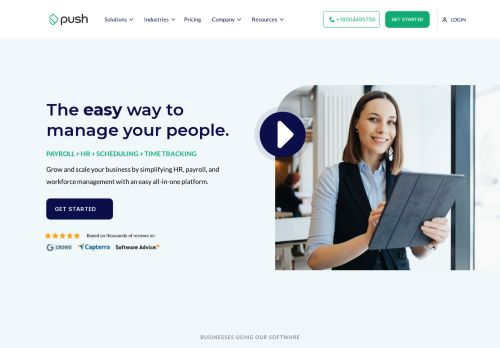This is a detailed caption for the described web page:

---

The web page for Push Industries showcases their employee management software. The page features a header with the company's name "Push" prominently displayed. Below the header, the tagline "The easy way to manage your people" is highlighted in blue over a light blue background. Adjacent to this tagline is a play button leading to an embedded video, likely providing an overview of their services.

The main section includes options for "Payroll," "HR," "Scheduling," and "Time Tracking," with these categories written in green text. Each option appears to be clickable, directing users to more detailed information. Beneath these options, there is a prominent blue button labeled "Get Started," encouraging visitors to sign up for the services.

Towards the bottom of the page, a single four or five-star review is visible, along with logos or mentions of partner companies or clients that Push Industries collaborates with. The footer includes a brief mention of the type of software offered, specifically business software, along with additional details.

Visually, the page also features an image of an elderly woman holding either a laptop or a tablet, which adds a personal touch to the otherwise business-centric web page design.

---